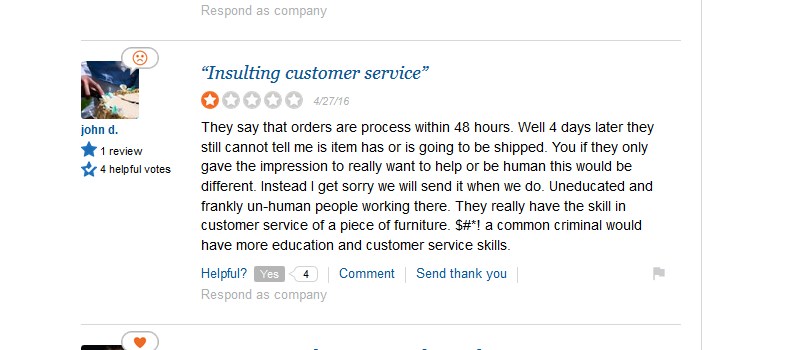This image is a landscape-oriented screenshot of a customer review from a website. The screenshot features a thin, vertical gray border on the right edge, set against a white background. At the top, there is gray text with an option to "Respond as Company." This text is separated from the review by a horizontal gray border.

The review section prominently displays a square avatar belonging to a user named John D, written in blue text. The avatar appears to be an image of some sand with a sad face text bubble coming from it. John D has written one review, indicated by a blue star, and has received four helpful votes, as shown by a blue star with a white checkmark.

The header of John D's review reads "Insulting Customer Service" in blue italic letters. He has given a rating of one star out of five, highlighted by an orange circle with a white star. The date of the review is noted as 04-27-16. 

In his review, John D criticizes the service he received. At the bottom of the review, there is a link that allows users to indicate if they found the review helpful, marked "Yes" with four tags next to it. Additional options include a "Comment" button and a "Send Thank You" button. Below this section, there is another option to respond as a company.